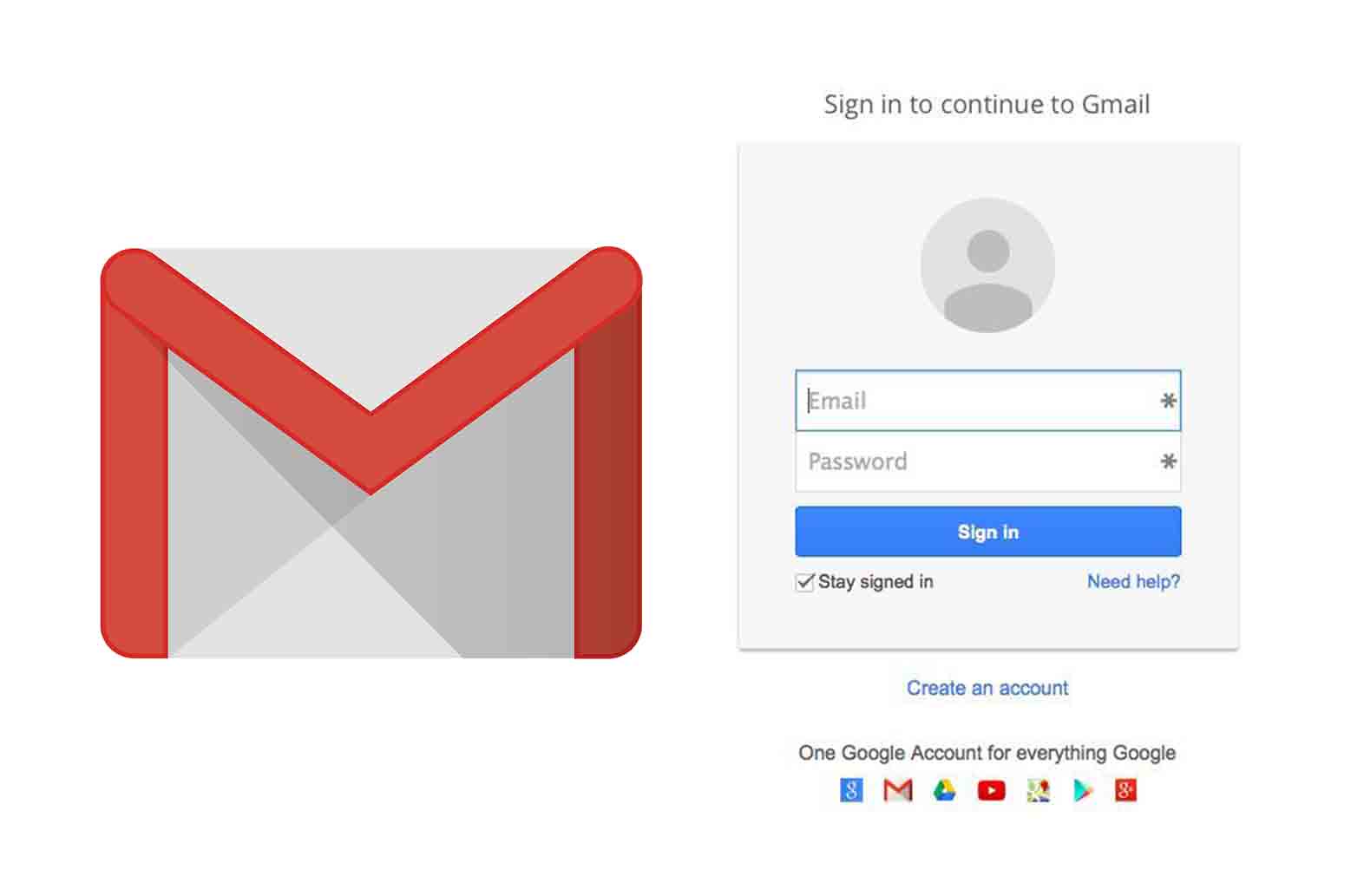Screenshot of the Gmail Sign-In Page

The image is a screenshot of the Gmail sign-in page. On the right side of the image is the iconic Gmail logo—depicted as a stylized envelope. The envelope's design incorporates an "M" shape formed by the red outer lines, with a white background filling the remainder of the envelope.

Adjacent to the logo is the login portal, which has a gray background. At the top of this section, centered, is a circular icon containing a simple, minimalist representation of a person—a circle for the head and a torso shape beneath it. Above this icon, in a neutral black font, is the text "Sign in to Gmail."

Below the person icon are two text fields. The first field, labeled "Email" with a red asterisk to indicate it is required, is highlighted in a bluish-green color. The second field, labeled "Password" with a similar red asterisk, appears below it.

Beneath the password field is a blue "Sign in" button, with the text "Sign in" in white. Under this button is a checkbox, which is marked, next to the text "Stay signed in."

To the left, there is a clickable "Need help?" link in blue text. Below this, there is an option to "Create an account," intended for users who do not yet have a Gmail account.

At the bottom of the sign-in portal is a statement: "One Google Account for everything Google," followed by various Google service icons. These include the Google logo, a mail icon, the Google Drive symbol, the YouTube logo, a maps icon, a blue triangle (indicative of Google Play), and a red icon whose specific service is not immediately clear.